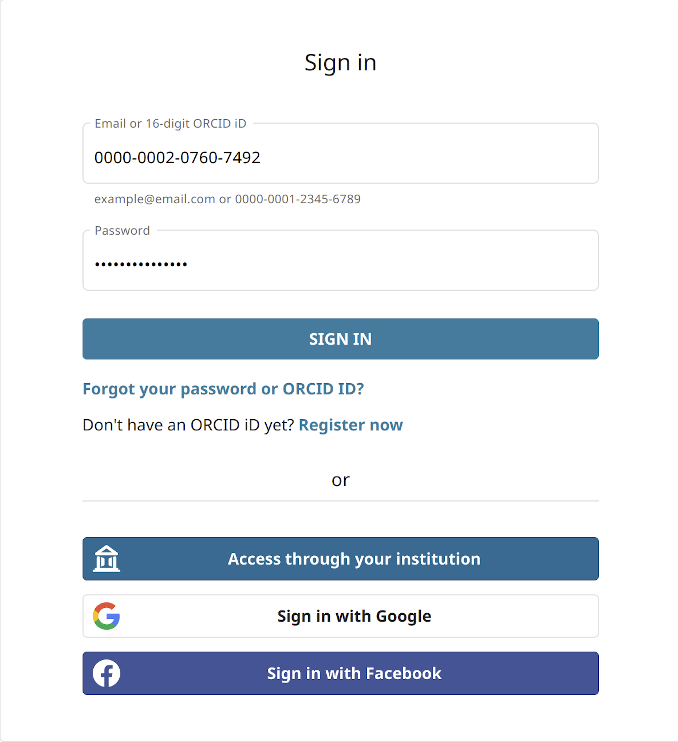This image captures the screen of a smartphone displaying a sign-in page. At the top of the page, the bold text "SIGN IN" is prominently featured. Below this heading, there is a long, slender white text box labeled "Email or 16-digit ORCID iD," which has been filled in with the number "0000-0002-0760-7492." Directly beneath this, there is a password entry field with obscured text indicating a long password has been entered.

Further down, a blue rectangular button with white, all-uppercase letters reads "SIGN IN." Below this button, there are additional helpful links: "Forgot your password or ORCID iD?" and "Don't have an ORCID iD yet? Register now." Following these links is a faint gray line with the text "or" splitting the line. The section below the line offers alternative sign-in options: "Access through your institution" depicted with a building icon, as well as buttons for "Sign in with Google" and "Sign in with Facebook."